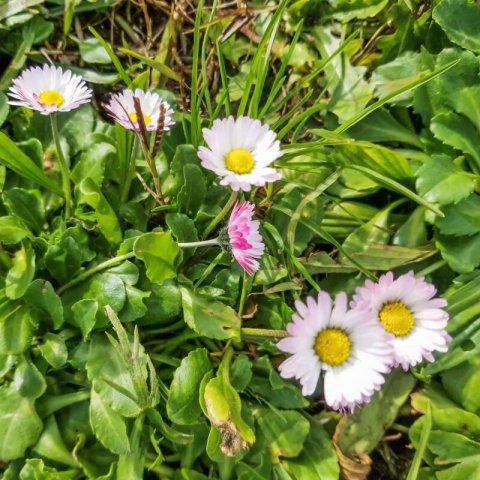The image showcases a close-up perspective of six delicate flowers, likely wildflowers or possibly daisies, nestled among lush green vegetation. The flowers exhibit white petals that transition to light pink or lavender hues toward the edges, with vibrant yellow centers housing the pollen. The scene suggests a naturally lit daytime shot, highlighting the vivid colors and various leaf textures surrounding the flowers. The backdrop includes leafy green vegetation with a mix of leaf types—some broad and flat, others spiny and narrow—and a few blades of tall grass. Notably, there are some brown leaves among the greenery, hinting at natural wild growth rather than a cultivated garden. One flower's back, which is more purple, is visible, providing a striking color contrast. The overall composition captures the beauty and complexity of these wild blooms against the rich, green, and slightly untended background of their environment.